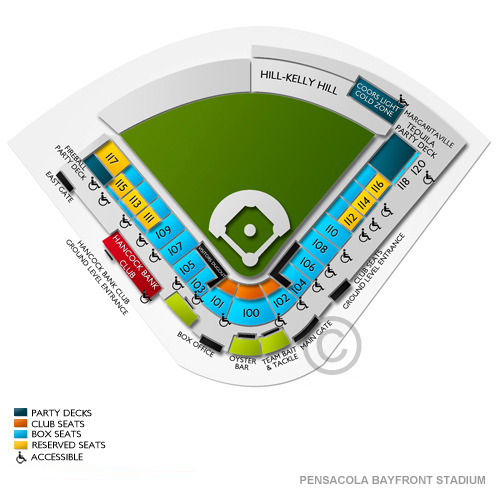This detailed map illustrates Pensacola Bayfront Stadium, depicted in the iconic triangular shape of a baseball field with one vertex pointing downward and the other two vertices positioned on the left and right sides. The background of the map is gray, providing contrast to the vivid details within the baseball field layout.

At the bottom of the map, the label "Pensacola Bayfront Stadium" is prominently displayed, and various streets and notable locations are highlighted. On the left-hand side, visitors can find the "Hancock Bank Club Ground Level Entrance," while the right-hand side features the "Club Seats Ground Level Entrance."

A striking red rectangle denotes the "Hancock Bank Club," positioned centrally on the map. Nearby, essential points of interest such as the box office, oyster bar, and team merchandise store "Team Bait and Tackle" are carefully indicated. The main gate and club section are also marked, ensuring ease of navigation for attendees. Multiple handicap accessibility icons are scattered across the map, emphasizing the stadium's efforts to accommodate all guests.

Surrounding the field, blue-colored box seats numbered from 100 to approximately 117 are labeled, suggesting prime seating areas for spectators. The baseball field itself is illustrated in green, complete with a clearly defined diamond at its center. True to form, the field emanates the charm and excitement typical of a traditional baseball stadium.

Adding a touch of whimsy and entertainment value, the map also features the "Margaritaville Tequila Party Deck," humorously named after a popular song. This playful detail adds to the overall appeal of the stadium, making it an inviting and lively venue for baseball fans and visitors alike.